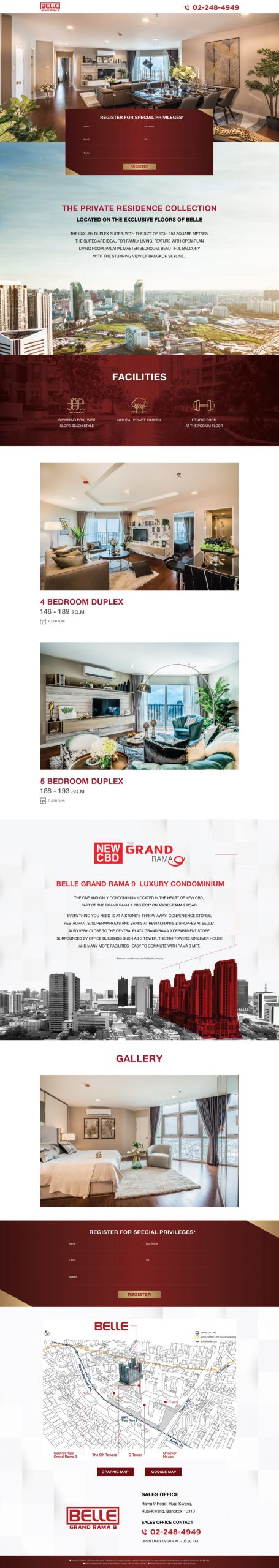The image is a blurry and distorted composition, making it challenging to discern the details clearly. In the upper section, there are several burgundy-colored boxes containing text. To the left of these text boxes, there appears to be an image depicting large hotels or houses adjacent to a grassy area. Below this, another burgundy text box is visible, followed by an image that seems to showcase the interior of a living room, possibly part of a hotel suite. The living room features a seating area, a television, and a large rug. 

Further down, the image stretches to reveal what appears to be a kitchen, identifiable by two large windows through which a blue outside setting is faintly visible. In the next section, a cluster of buildings is showcased, with those on the right being red and those on the left being gray. 

Following this is an image of a spacious bedroom with tall, open windows adorned with gray curtains. The bed in this room is covered with beige blankets, and the walls are painted a tan color. Below this bedroom image lies another burgundy-colored rectangle. The final section of the image seems to display a map, characterized by numerous gray lines crisscrossing throughout.